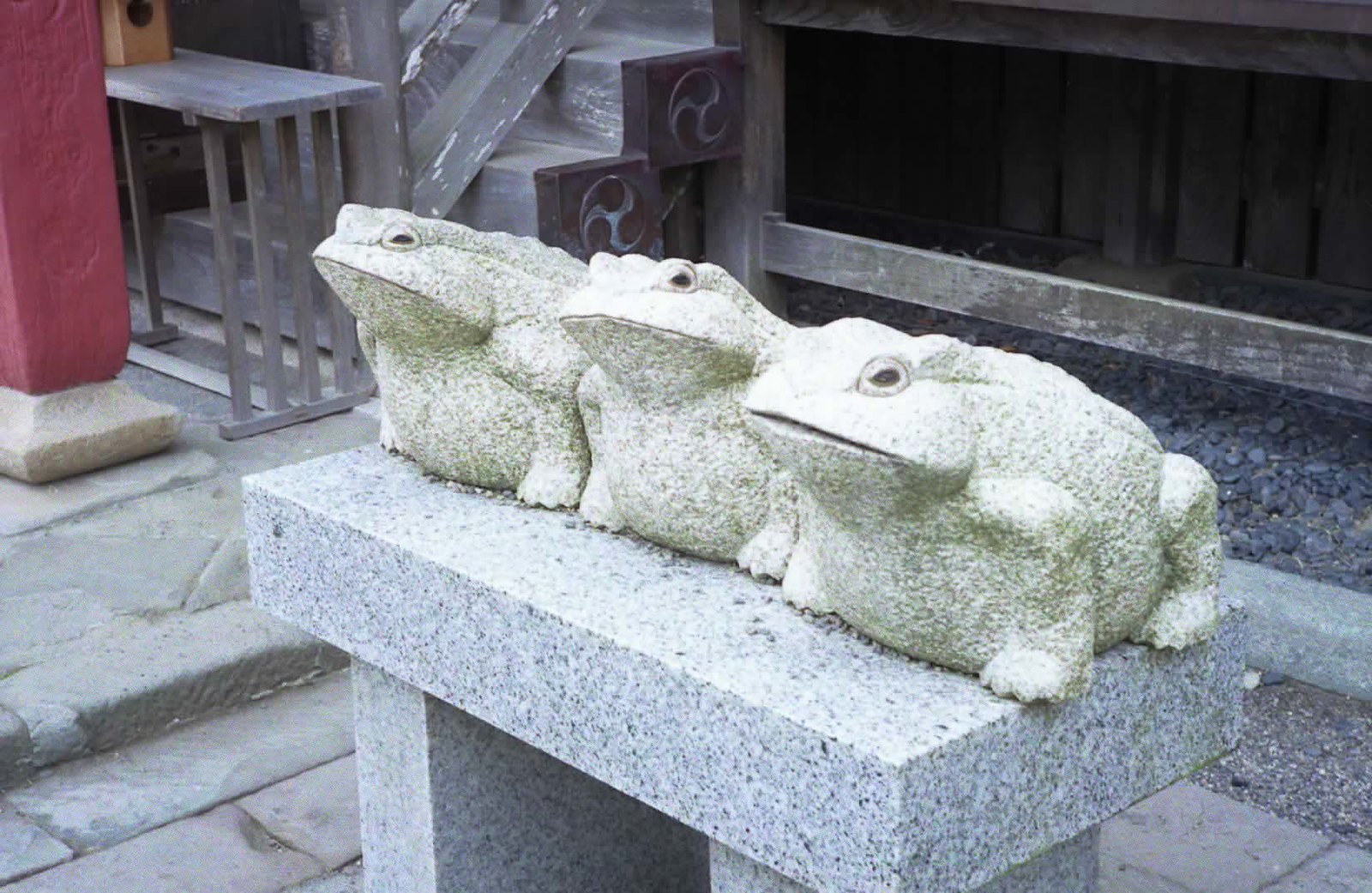The image features a handcrafted sculpture of three white stone bullfrogs, resembling garden decor. These plump amphibians, with black beady slit-like eyes, sit in unison on a stone bench atop brick and mortar tiles. The frogs face slightly left, revealing their left eyes and mouths, with faint details of scales on their backs and their front feet visible. Behind the stone bench, to the left, there is a wooden bench beside a red column, and wooden stairs with decorative detailing lead up to what appears to be a porch area. The setting is outside, with loose gravel underneath the porch, creating a quaint garden-like atmosphere.